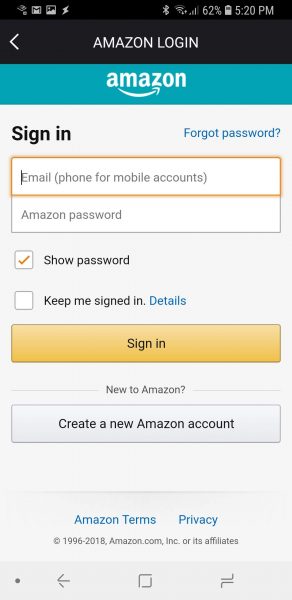This detailed, cleaned up caption describes an Amazon login screen captured from a mobile device:

---

The image displays an Amazon login page, as seen on a tablet or smartphone. At the top, several icons are visible: an unrecognized symbol, followed by icons for Gmail, screenshots, and a low battery indicator. On the right side, the status bar shows a Bluetooth symbol, a nearly full WiFi signal icon, and a similarly strong cell phone signal indicator. Next to these, "62%" denotes the remaining battery life, followed by the time reading 5:20 PM.

Beneath this, a black bezel features "Amazon Login" in white text on the left, accompanied by a white arrow. Below this, a cyan blue bar displays the Amazon logo, with an arrow stretching from 'A' to 'Z'. 

The login section begins with "Sign-In" in bold black text on the left and "Forgot password?" in blue, hyperlinked text on the right. Below, two gray rectangles indicate the input fields; the first one is selected, indicated by an orange border and a blinking cursor. The placeholder text in this field reads "Email (phone for mobile accounts)".

Below, the password field is also indicated in a gray rectangle, with two checkboxes below it. The first checkbox, labeled "Show password" in bold black, is ticked with an orange checkmark. The second checkbox, labeled "Keep me signed in", is unchecked, with "Details" as hyperlinked text in blue beneath it.

The "Sign-In" button is prominently placed below these fields, in orange-yellow with black text. Further down, the page asks "New to Amazon?" in gray text followed by a gray button labeled "Create a new Amazon account".

At the bottom, "Amazon Terms and Privacy" is written in hyperlinked blue text. Beneath, the copyright notice reads "Copyright 1996-2018, Amazon.com, Inc. or its affiliates", indicating the screenshot is from 2018.

The bottom bezel of the device is dark gray, featuring navigation icons including a dot, a back arrow, a square for the home button, and two overlapping L's.

---

This caption provides a detailed and clear description of the Amazon login screen, making it easily understandable for someone who has not seen the image.